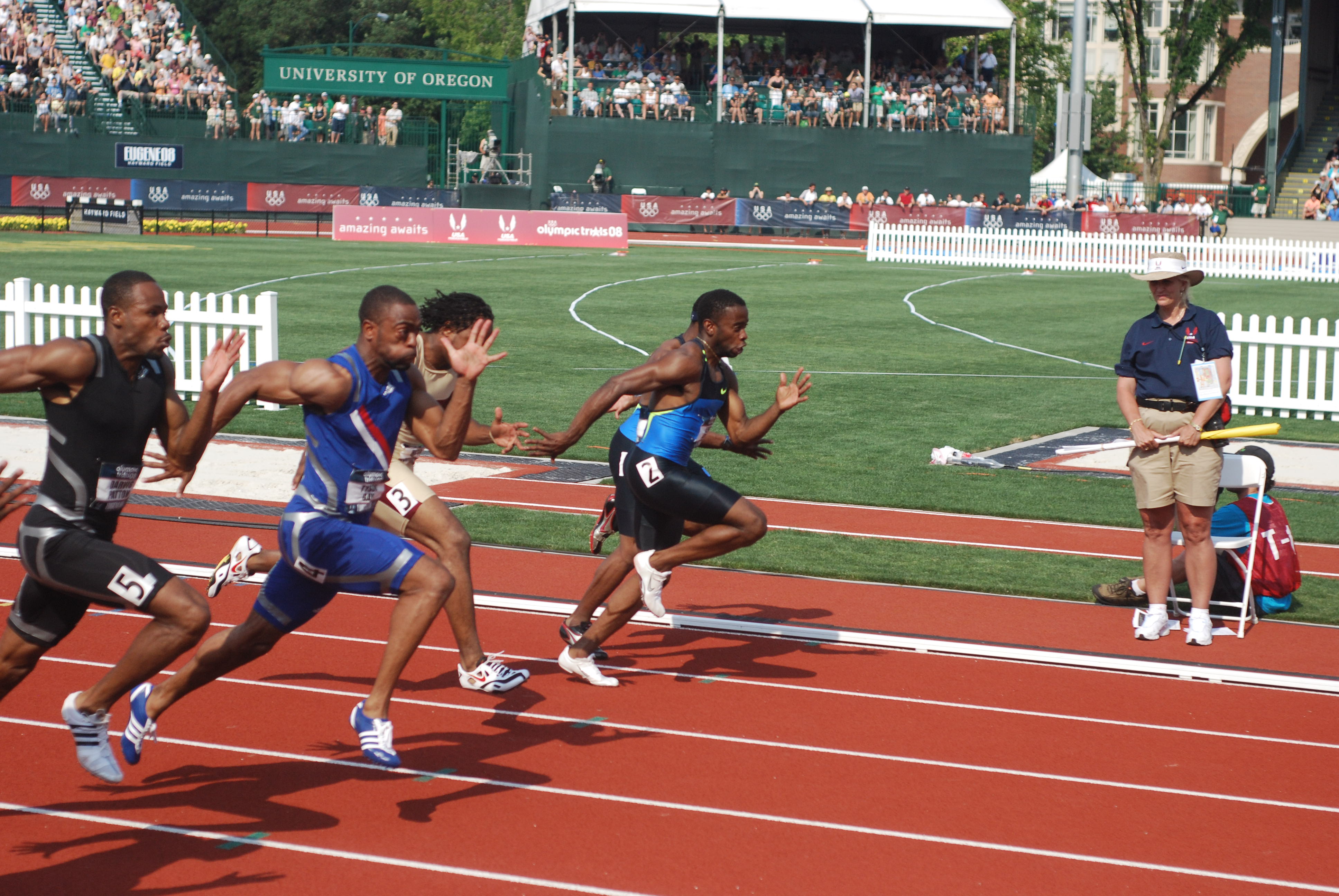The image captures an exhilarating track race featuring a group of African American athletes, all running on a red track field. The runners are clad in various outfits: one in all black with the number five, another in blue and red stripes, one in a beige tracksuit, and two in black and blue uniforms. They are all in mid-stride, legs up, as they compete. To the left, there is a glimpse of another person's fingers in the frame.

Off to the side stands a race official, dressed in a navy blue polo shirt, khaki shorts, white sneakers, and a sun hat, possibly serving as a timekeeper or judge. Behind him, a person sits on the grass. In the background, the image prominently features a sign that reads "University of Oregon" in white capital letters against a green backdrop, suggesting the location is likely Hayward Field. Beyond the sign, a lush green field is fenced off by a white picket fence, and the stands are packed with spectators, eagerly watching and cheering the runners on.